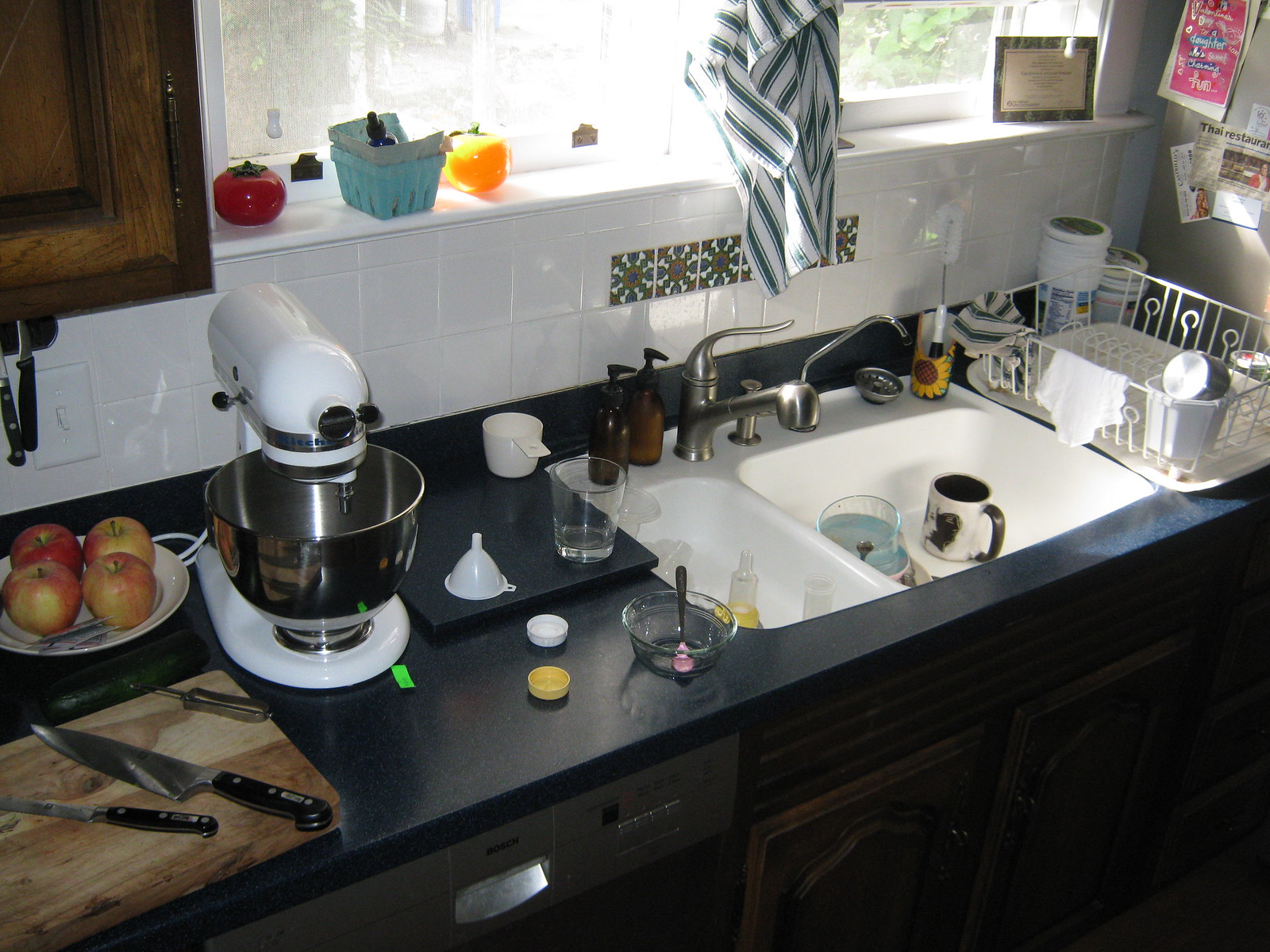This detailed landscape-style image captures a kitchen scene with a double window at the top, adorned with a tomato crate, an orange case, and a blue container. A green and white striped towel hangs prominently in the center of the image. To the top left, there is a partially visible cabinet due to the image's margins.

The kitchen features a white tiled backsplash, beneath which, on the left middle side of the image, rests a white plate with four red apples. In front of the plate is a brown cutting board holding a butcher knife, a smaller knife, and a paring knife. These items sit on a sleek black granite countertop. 

Next to the apples, on the right, is a mixer with a stainless steel bowl and a white mixing base. Further to the right, a glass cup is positioned near a full white sink containing several mugs with white and brown handles. The sink has a stainless steel faucet and is flanked by two brown soap bottles. An empty white rack is situated to the immediate right of the sink, completing the composition.